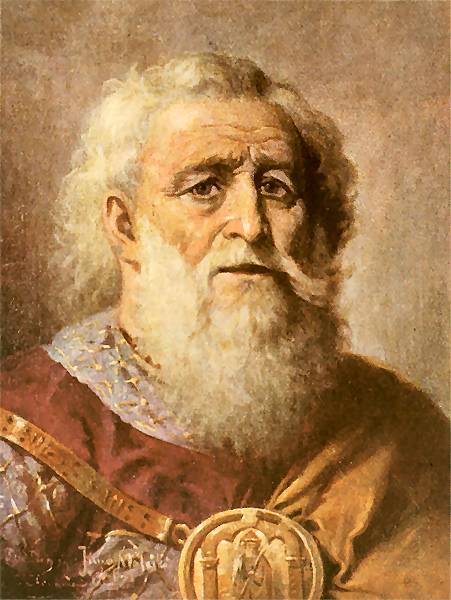This detailed color oil painting, titled "Mieczko the Old," by artist John Matejko (M-A-T-E-J-K-O), is a striking Romanticism portrait rendered in portrait orientation. The subject is an elderly man, possibly in his late 80s or 90s, with a long white beard and mustache, and long white hair parted in the middle. His expressive hazel eyes convey a sense of worry and concern. The man is depicted as a regal figure, potentially a general warrior or a king, dressed in elaborate attire. He wears a robe adorned with a luxurious gold cloth draped over his left shoulder and a russet collar with a gold band, over a light blue or greyish-blue garment detailed with gold accents. His outfit includes a golden round medallion on his chest, depicting a saintly figure standing between two columns, which is attached by a chain. The background comprises predominantly brown and beige brush strokes, complementing the warm, earthy tones of the clothing and enhancing the aura of the painting.